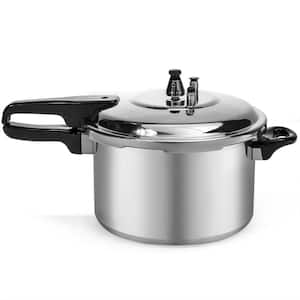This is a highly detailed, color product image of a substantial stainless steel pressure cooker resting on a white background, with no visible borders. The pot itself is silvery metallic, with a shiny top lid indicative of stainless steel and a brushed aluminum appearance on the bottom. It features two black plastic handles: a short, regular handle on the right meant for lifting, and a longer handle on the left that doubles as a way to rotate and secure the lid. This lid, which is transparent, has a small black triangular handle for easy removal. The top of the pressure cooker is outfitted with pressure relief valves that regulate steam release during cooking. The overall design includes functional and safety elements like gaskets to maintain the cooker under pressure. The cooker is well over a quart in volume, suggesting it’s designed for cooking substantial quantities of food like potatoes and various vegetables.